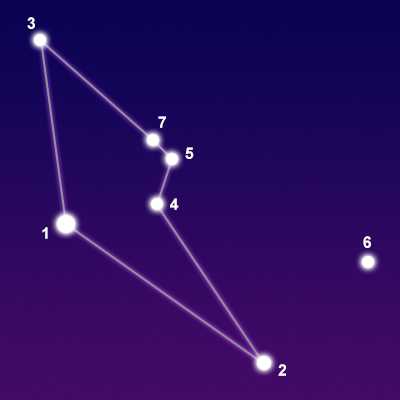The image appears to be a detailed diagram or illustration, possibly depicting a constellation against a varied background. The backdrop transitions from a deep purple at the top to a lighter purple at the bottom, with a dark blue hue on the top left gradually blending into the purplish tones on the bottom right. In the forefront, there are seven bright white lights, each numbered from 1 to 7. These lights vary in size, with some appearing smaller and others slightly larger. They are arranged in a non-sequential pattern, connected by light purple lines forming a zigzag or lightning bolt shape that links dots 1, 2, 4, 5, 7, and 3. Dot 6 is positioned separately to the far right and is not connected by any lines, standing alone amidst the pattern.